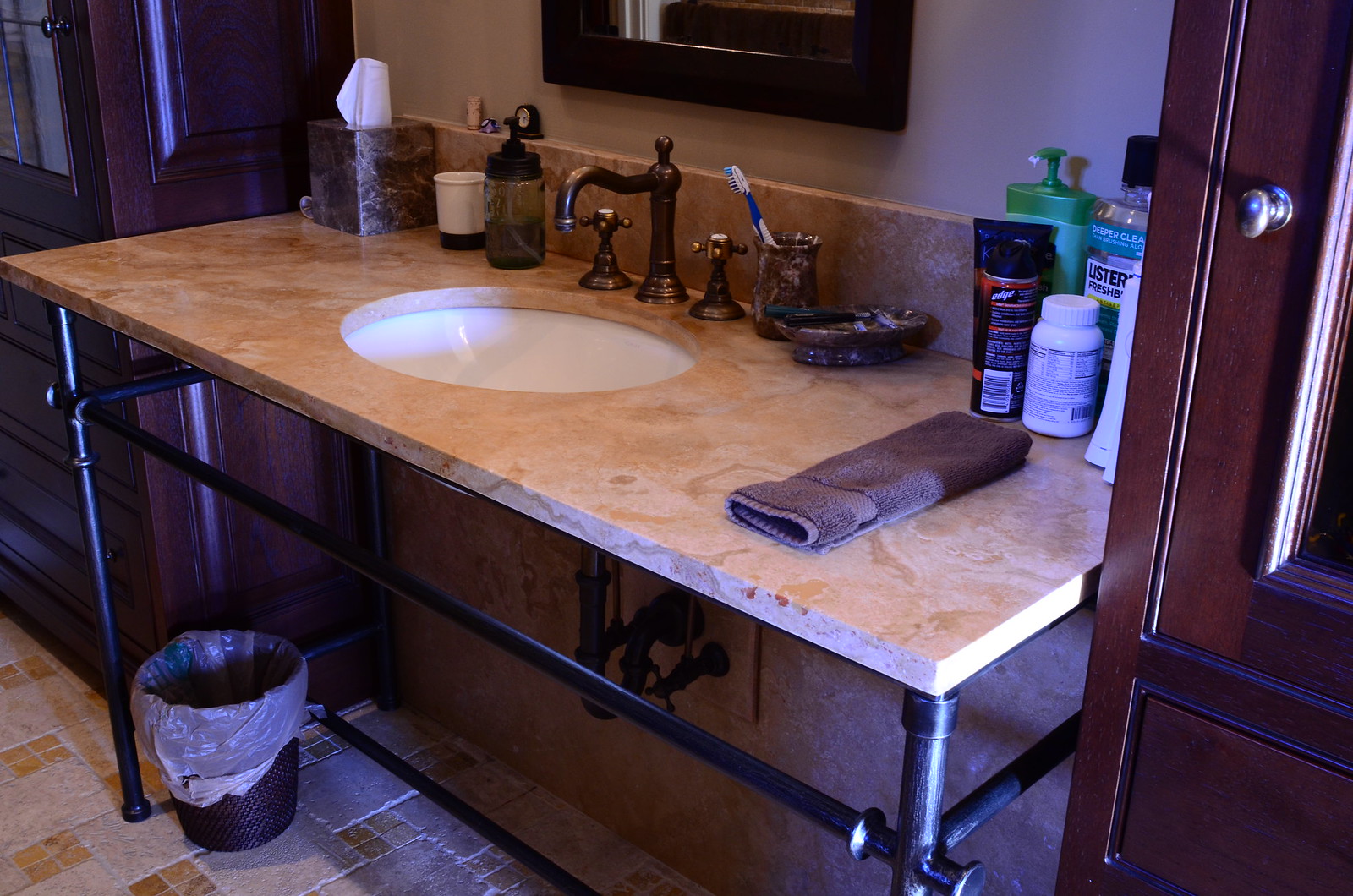The image portrays a bathroom counter with a light brown surface. Centrally positioned is a white porcelain sink with a short, copper-colored faucet. Accompanying the main faucet are two smaller turn-style handles for adjusting water temperature. To the right of the sink, there's a small cup holding a toothbrush, and further right, various bathroom items can be seen: shaving cream, a small white pill bottle, a tall green lotion bottle, and a bottle of Listerine mouthwash. A neatly folded brown towel is placed in the right corner, near the partly visible brown door with silver hardware. On the left side of the faucet, there is another white cup and a brown tissue holder with a white tissue protruding from the top. The floor is tiled in brown, and a small black wastebasket with a liner is situated at the bottom of the image.